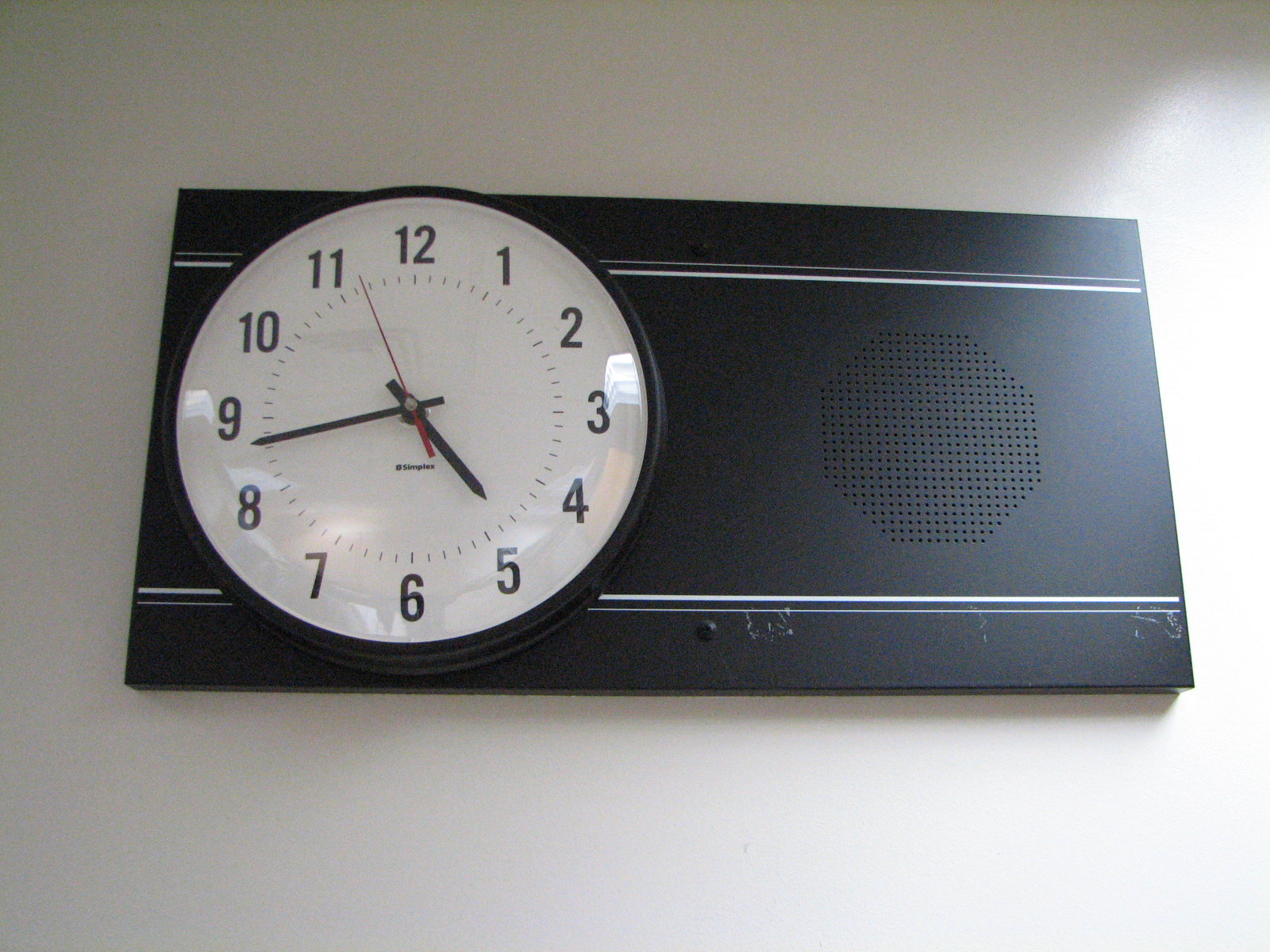The image showcases a wall-mounted clock set against a white backdrop. The clock is secured on a black base adorned with white stripes. Adjacent to the left side of this base is a hexagon-shaped speaker, characterized by tiny perforations in its plastic surface. The clock itself is circular and prominently featured beside the speaker. The clock's exterior casing is a sleek black, while its interior face is a stark contrast in white. Black numerals mark the hours, with the minute and hour hands also in black, both tapering to pointed ends. The second hand provides a striking accent in red, standing out against the monochrome palette of the clock face.